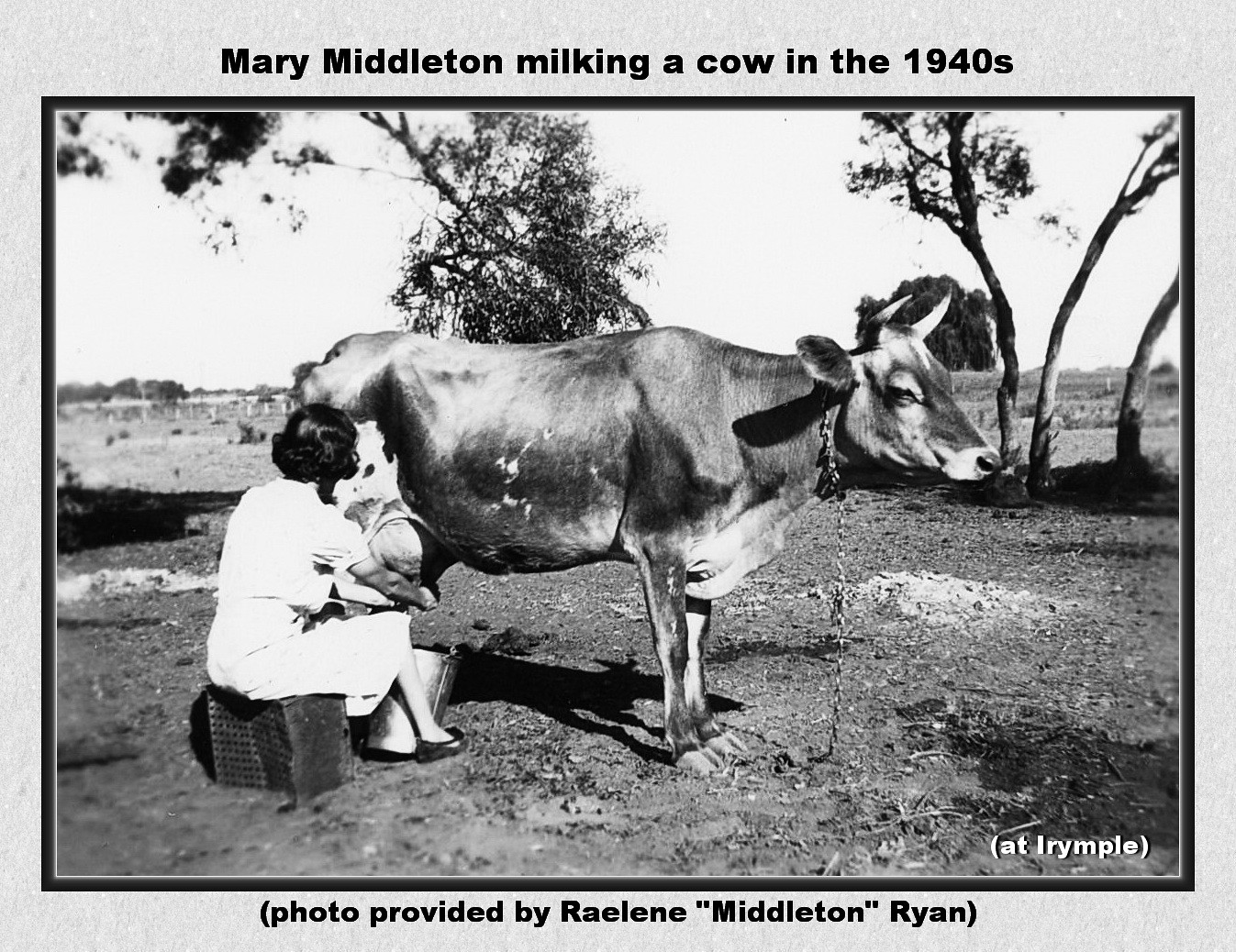This black and white photograph, likely the front side of a postcard bordered by a black line, captures Mary Middleton in the 1940s milking a cow. The image features a woman, wearing a white dress typical of the era and having short brown hair, sitting on a small wooden or milk crate stool. She is milking a cow, possibly a bull given its horns, into a metal bucket. The cow has a chain hanging around its neck. The scene is set outdoors in a field with some bare dirt and spindly sapling trees in the background. Surrounding the photograph is a gray border where the top edge reads, "Mary Middleton milking a cow in the 1940s," and at the bottom, it says in smaller text, "photo provided by Raylene Middleton-Ryan." The overall appearance suggests an archival quality, evoking a sense of nostalgia from the mid-20th century.